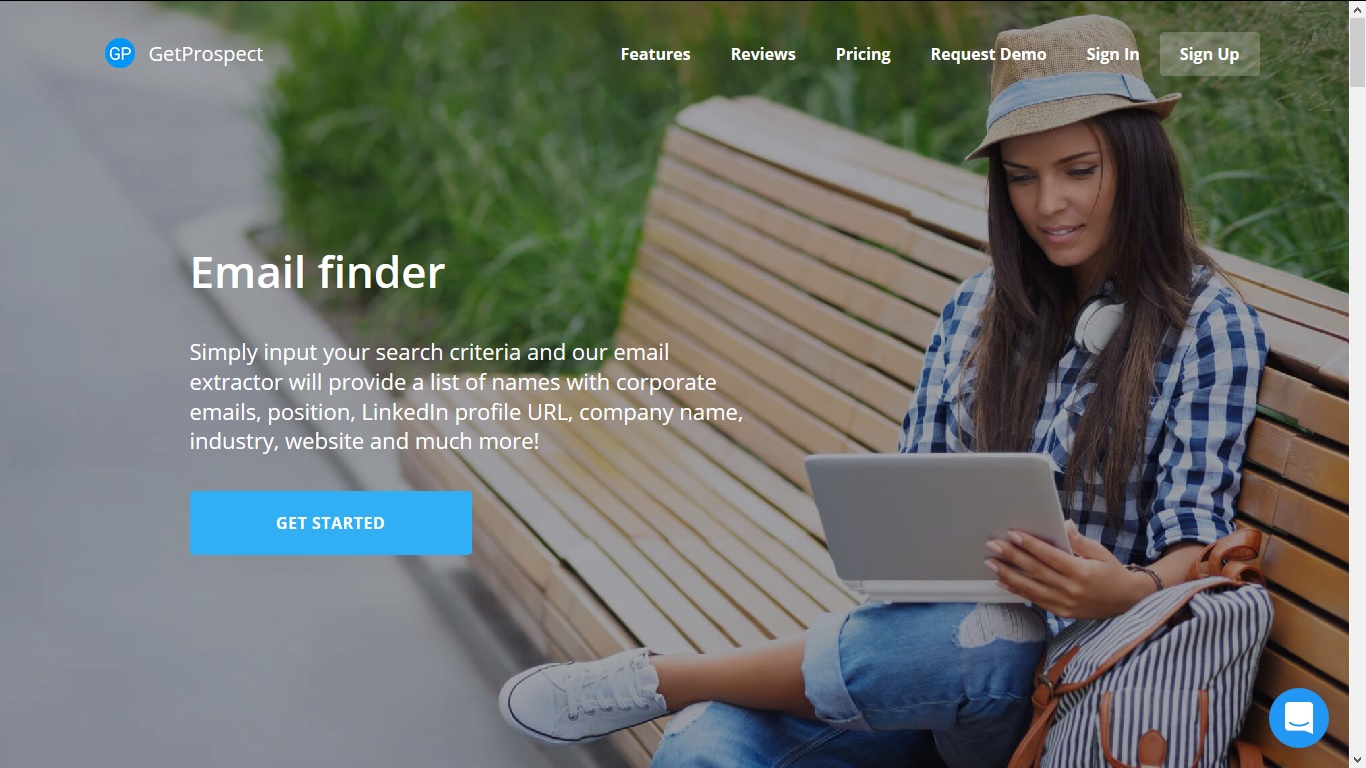This image, captured from a smartphone web page, displays the homepage of "Get Prospect." At the top of the screen, a blue circle contains the initials "GP" next to the website's name. The navigation bar includes menu options: Features, Reviews, Pricing, Request Demo, Sign In, and Sign Up. Centrally featured is a prominent section titled "Email Finder" with an invitation to input search criteria for the email extractor, which promises to return names with corporate emails, LinkedIn profile URLs, company names, industries, websites, and more. Beneath this, a blue "Get Started" button with white text is prominently displayed.

In the foreground, a woman sits on a bench with a Chromebook or tablet on her lap, engrossed in reading. She wears a beige hat accented with a blue stripe, a white and blue plaid shirt, light blue jeans, and white shoes. The backdrop consists of tall grass, suggesting an outdoor setting.